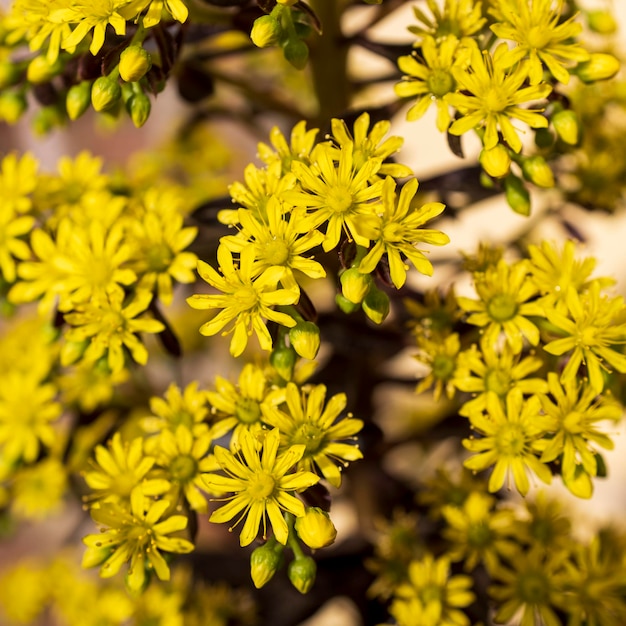The image depicts a close-up view of vibrant yellow flowers, clustered together against a blurred background to emphasize their vivid details. Each small flower, approximately the size of a nickel, features around 9 to 10 petals radiating outward from a central greenish-yellow cluster of seeds, giving the flowers a sun-like appearance. The majority of the flowers are in full bloom, while several buds in the upper left-hand corner are just beginning to open. The flowers are grouped in clusters along brown branches, accompanied by small green buds and highlighted by subtle hues of yellow and white from light filtering through the background. The overall composition focuses keenly on the yellow flowers, enhancing their beauty and intricate details against the softly out-of-focus backdrop.